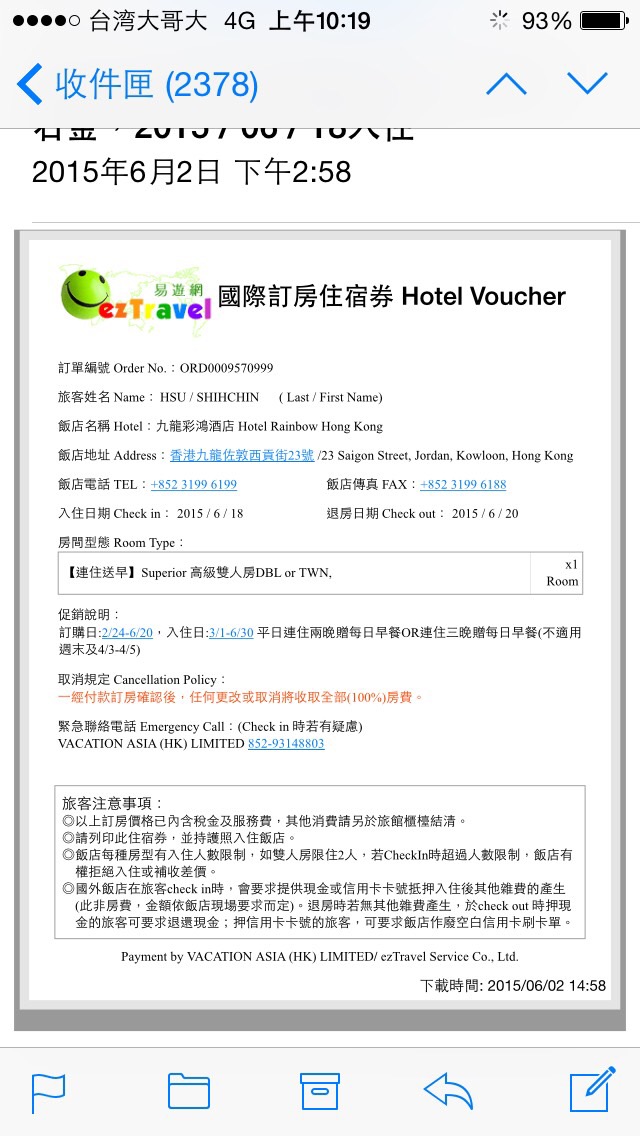This detailed and descriptive caption unifies the provided information:

"This is a screenshot taken from a mobile phone, likely an iOS device, displaying an email inbox. The email in focus is mostly written in Chinese and presents a hotel voucher from EasyTravel. At the top of the email is the EasyTravel logo, featuring a colorful design and a tennis ball with a smiley face. Right next to the logo, the text reads 'Hotel Voucher,' with a small map highlighting China. The email is essentially a receipt detailing the hotel stay, including order number, guest name, hotel address, telephone number, fax number, check-in time, checkout time, room type, cancellation policy, and emergency numbers. There are options at the very bottom of the screen to reply, forward, or archive the message. The phone's battery status shows 93% at the top of the display."